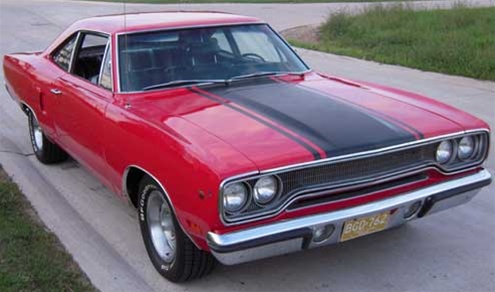The image captures a striking red classic muscle car, possibly from the 1970s, adorned with a bold black racing stripe down the center of the hood, flanked by two thinner black stripes. The interior features black seats and a black steering wheel, with the left passenger window rolled down. The car is parked on a pale gray driveway extending onto a darker concrete road. A silver bumper and grill highlight the front, accompanied by unlit white headlights. A yellowish license plate reads BGO-762, though specifics about the state remain unclear. Flanking the vehicle are green grass yards, situating it in a daytime setting with clear visibility of surrounding paved streets and curving paths. The silver rims and black tires complete the distinctive appearance of this vintage automobile.